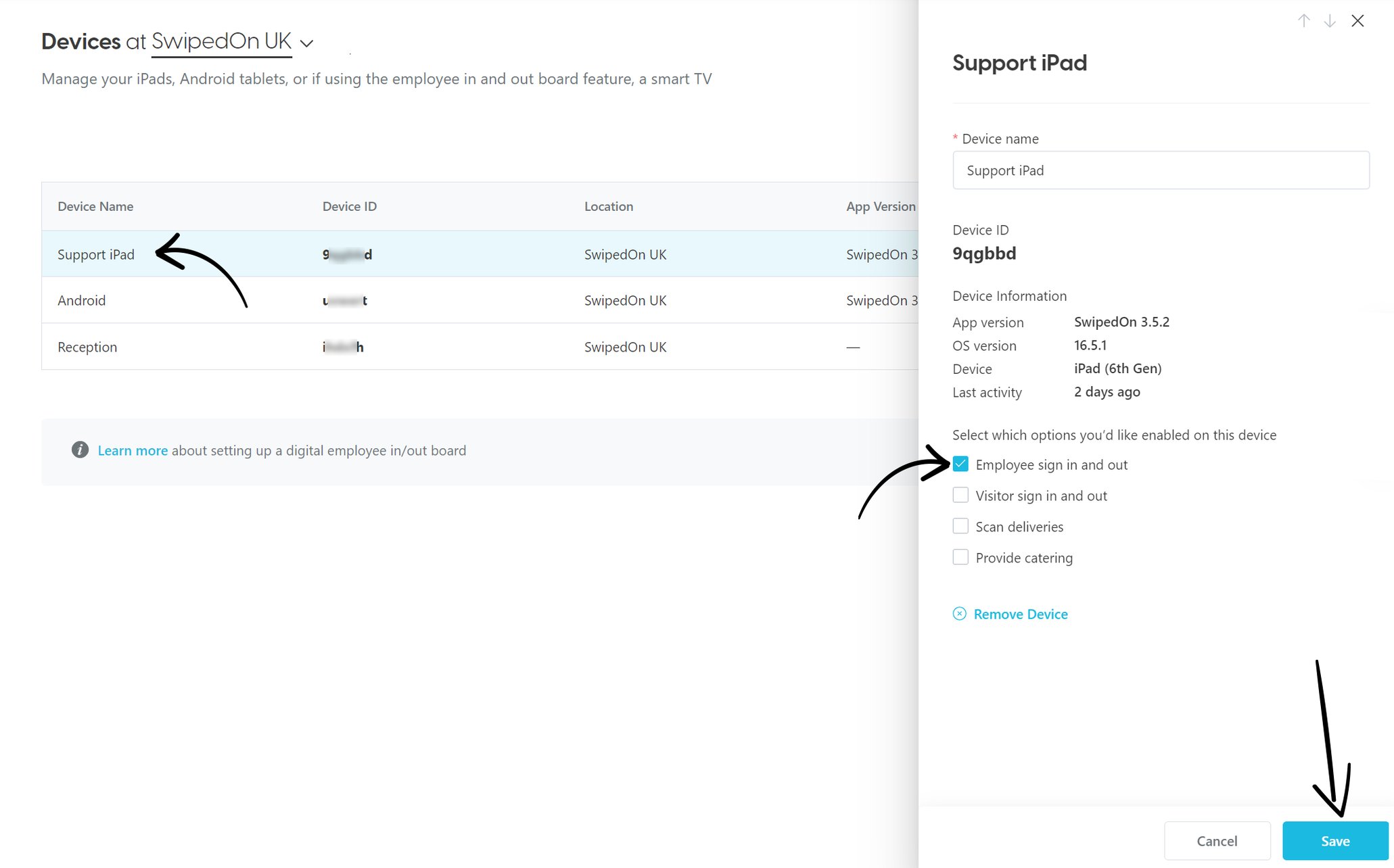The image depicts a specific page on a website designed for managing devices under the SwipedOn UK platform. The page features a clean white background with the content primarily aligned to the left.

On the left side of the page, the text "Devices at SwipedOn UK" is prominently displayed, followed by a dropdown menu. This menu provides the options to manage various devices including iPads, Android tablets, and smart TVs if the Employee In and Outboard feature is being used.

Below this dropdown menu, there are four fields arranged in a vertical list: Device Name, Device ID, Location, and App Version. Each field is populated with specific details:

1. **Support iPad**
   - **Device ID:** Blurred
   - **Location:** SwipedOn UK
   - Notably, the "Support iPad" has a black arrow pointing to it and is highlighted in light blue instead of white.

2. **Android**
   - **Device ID:** Blurred
   - **Location:** SwipedOn UK

3. **Reception**
   - **Device ID:** Blurred
   - **Location:** SwipedOn UK

Underneath these fields, there is a prompt to "Learn more about setting up Digital Employee In and Outboard."

On the right side of the page, detailed information about the "Support iPad" is provided:
- **Device Name:** Support iPad
- **Device ID:** 9QGBBD
- **Device Information:**
  - **App Version:** SwipedOn 3.5.2
  - **OS Version:** 16.5.1
  - **Device:** iPad, 6th Generation
  - **Last Activity:** 2 Days Ago

Following this, there is an option to "Select which options you would like to enable on this board," with "Employee Sign In and Out" being one of the enabled options, indicated by another arrow.